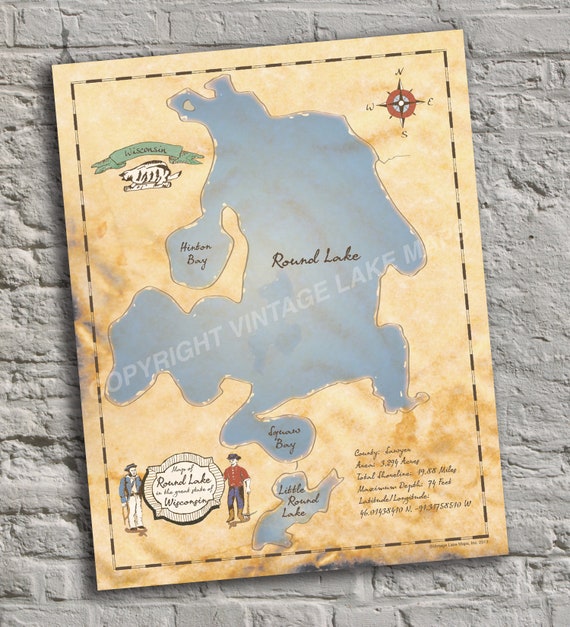The promotional image features a vintage-styled, hand-drawn poster of a map labeled "Round Lake" against a distinctive white-painted brick wall background. The wall, which has been covered with plaster in patches, shows areas where the plaster has come off, exposing the underlying texture. The rectangular poster, oriented in portrait and slightly tilted with its bottom left corner lower than its top right, measures twice as long in width compared to its height. The map's background is cream-colored, with a light blue, irregularly shaped lake positioned in the center top. Prominent annotations include "Round Lake" in black script on the right, "Hudson Bay" on the left, and "Little Round Lake." Additionally, a green banner with illegible text is above "Hudson Bay," and a compass rose indicating the cardinal directions is located in the top right. The bottom left corner of the poster features illustrations of two men in vintage uniforms standing on either side of a white shield that reads "Map of Round Lake." The poster has been given a burnt texture on the bottom and left edges, contributing to its aged appearance. The overall style of the image is a blend of photographic realism and representationalism.